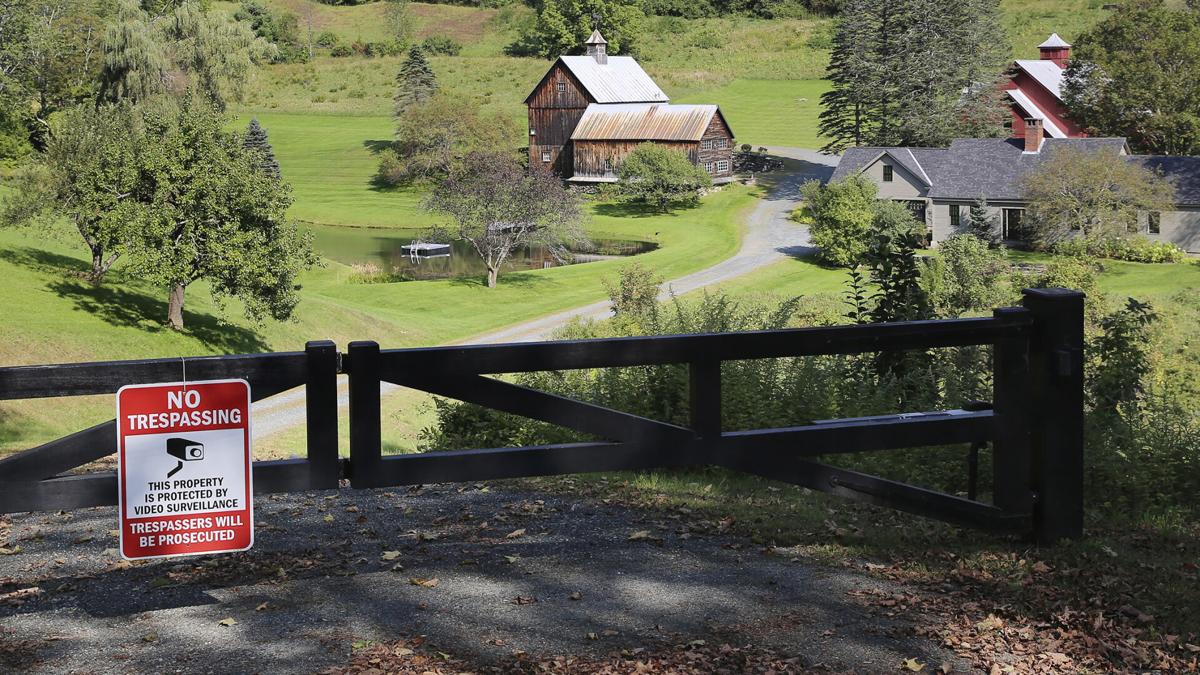The image depicts a serene rural homestead viewed from a hill. In the foreground, a black iron gate spans from left to right, prominently featuring a red and white sign that reads, "No Trespassing. This property is protected by video surveillance. Trespassers will be prosecuted," accompanied by a camera icon. The ground at the gate is paved and scattered with clumps of leaves. 

Beyond the gate, a gravel driveway curves down the hill, flanked by lush greenery and clumps of trees, leading to several structures. To the left of the driveway, a picturesque pond surrounded by trees features a floating raft. Dominating the view is a large rustic wooden barn with a tin roof and a central stack, giving it an almost mill-like appearance.

Adjacent to the barn, there is another horizontally shaped barn, and across the driveway stands a ranch-style gray house with a brick chimney and a dark gray roof. In the distance, partially visible behind these main buildings, is the roof of a red barn with a tin roof. The background is dotted with trees scattered across rolling grassy fields, with more hills and trees extending into the horizon. The scene is bathed in sunlight, enhancing the homestead's peaceful and idyllic atmosphere.